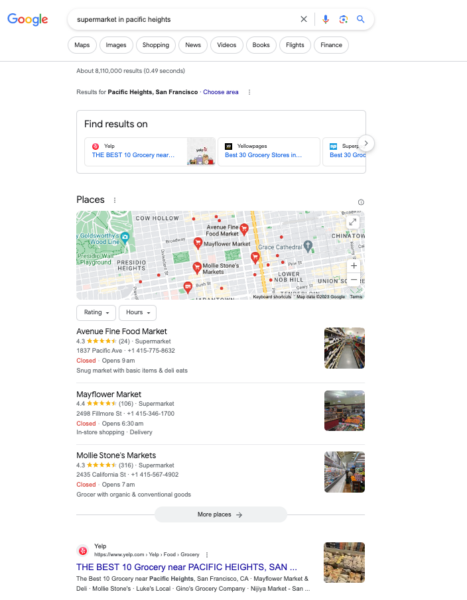A detailed screenshot depicting a Google search for "supermarkets in Pacific Heights" on a mobile phone. At the top, there's a search bar with the query "supermarket Pacific Heights." Below it, Google provides various filtering options: maps, images, shopping, news, videos, books, flights, and finance.

The search results title reads "Results for Pacific Heights, San Francisco," with a rectangular prompt directing users to find results on Yelp and Yellow Pages. Below this prompt is another rectangle labeled "Places," containing a map with several pin drops indicating locations of interest. Three specific supermarkets are prominently featured:

1. **Avenue Fine Food Market** - Rated 4.3 stars and currently closed. To the right, there is an image depicting grocery store aisles.
   
2. **Mayflower Market** - Rated 4.4 stars and also currently closed. The accompanying image shows the store interior.

3. **Mollie Stone's Markets** - Rated 4.3 stars, this one is similarly closed at the moment. An image to the right illustrates a shopping aisle.

At the bottom of the screen, a Yelp result highlights "The Best 10 Grocery Stores near Pacific Heights."